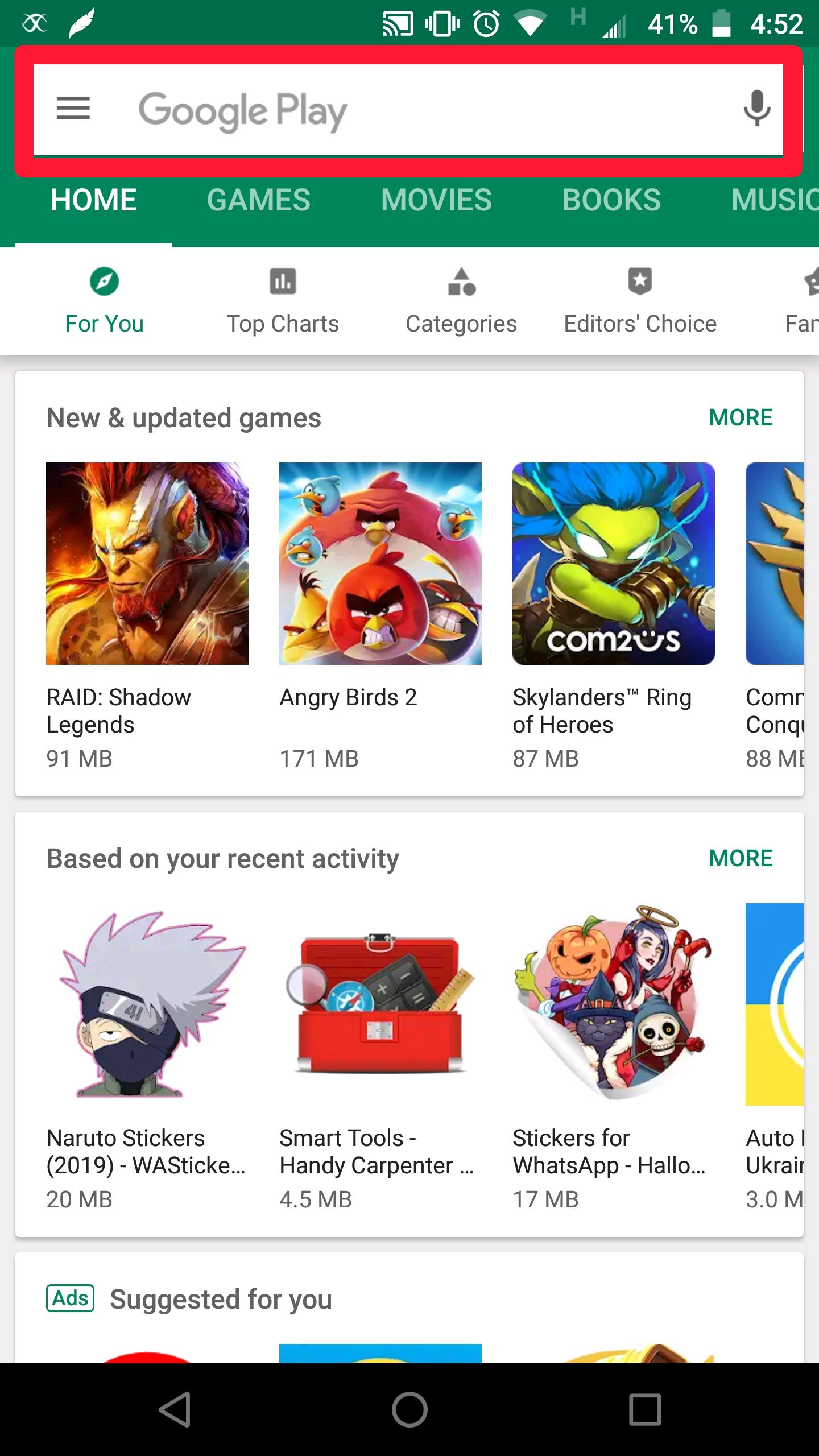The screenshot is from the Google Play Store displayed on a mobile device. The top section features a red box highlighting the search bar, which displays "Google Play" and includes a microphone icon to its right. Below the search bar, there are navigation tabs labeled as Home, Games, Movies, Books, and Music.

Further down, a secondary navigation bar is visible with categories For You, Top Charts, Categories, Editors' Choice, and another partially cropped tab, likely "Family." 

The primary content area showcases a box titled "New and Updated Games" on the left, with "More" in green text on the right. The games listed include:

1. **Raid: Shadow Legends** - 91 MB, featuring an image of an angry orc warrior looking down.
2. **Angry Birds 2** - 171 MB, represented by several furious birds.
3. **Skylanders™ Ring of Heroes** - 87 MB, displaying a goblin with blue hair, glowing white eyes, and wearing gauntlets. The developer, Com2Us, is mentioned underneath.

Another section labeled "Based on Your Recent Activity," also with a "More" option, lists additional apps:

1. **Naruto Stickers 2019 - WAStickers** - 20 MB, which shows an image of Kakashi from the Naruto series.
2. **Smart Tools: Handy Carpenter** - 4.5 MB, depicted by a toolbox containing a compass and ruler.
3. **Stickers for WhatsApp: Holo** - 17 MB, featuring characters such as a goblin, jack-o'-lantern, skeleton, and a witch cat.

The detailed layout and images provide a clear overview of various game recommendations and utility tools available on the platform.